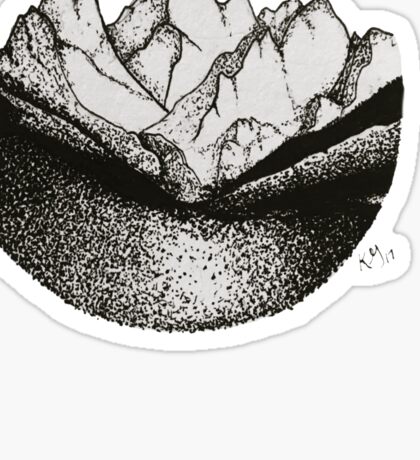This photograph features a partially cropped, stylized patch or sticker with a light gray background. The patch is mostly round, with a small nub on the bottom right showcasing the artist's autograph, which reads "KY17," likely indicating the year 2017. The artwork on the patch, executed in black ink, consists of intricate dot and line patterns. The drawing depicts a semi-circular valley leading up to a jagged mountain range comprising five to six peaks. The mountaintops are white, contoured by the top edge of the patch. The lower part of the image features densely packed black dots that create a textured appearance, possibly mimicking grass or a waterway, gradually dispersing to reveal the gray background. The overall design blends solid black, sparse dots, and shading to produce a compelling black-and-white sketch.